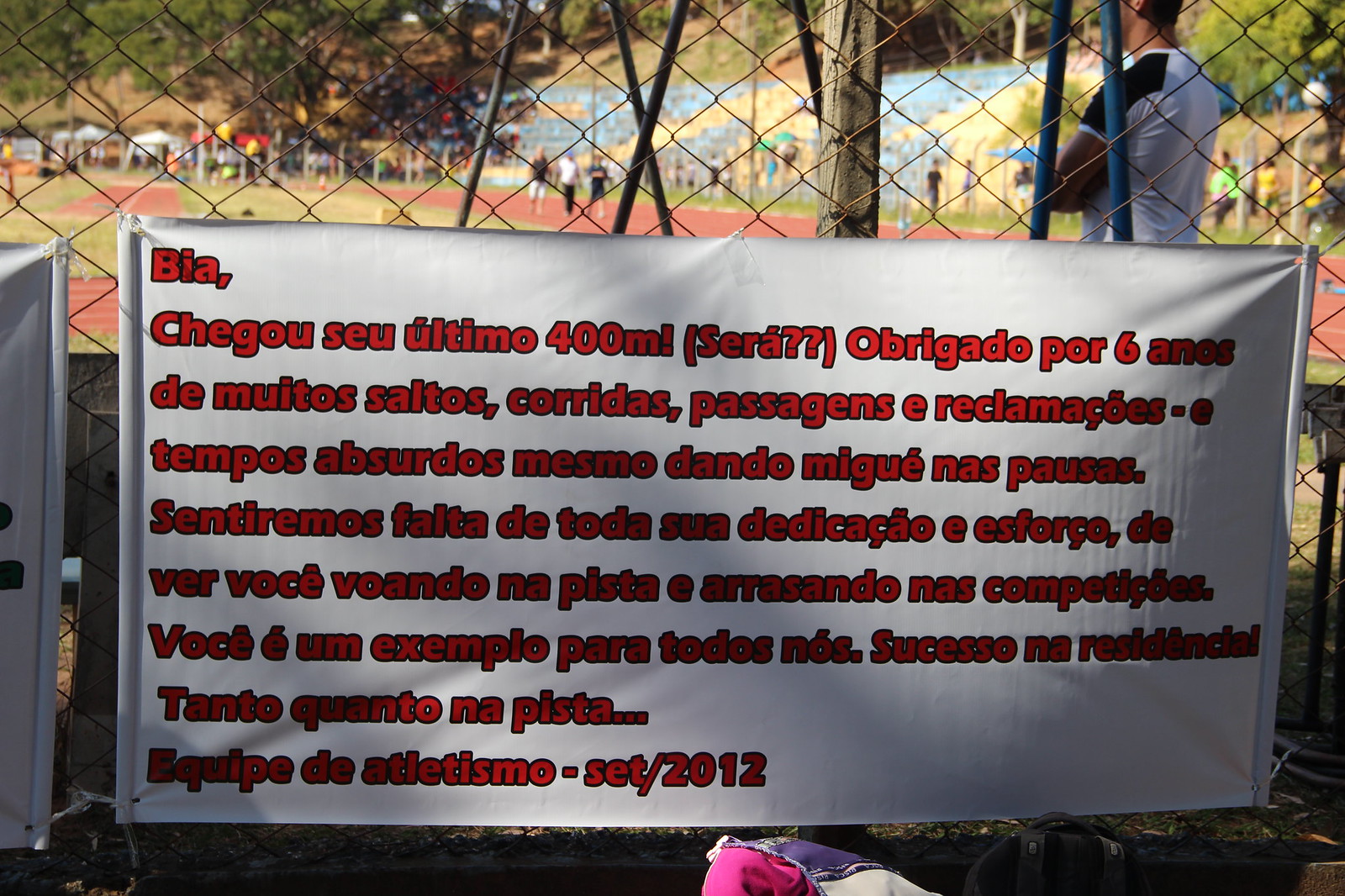This photograph captures a vibrant scene centered around a baseball or softball game. The image is slightly wider than it is tall, featuring a prominent sign occupying about 75% of the horizontal space, stretching from roughly 10% to 90% across the frame. The sign, attached to a chain link fence, is white with text in bright red—which appears to be either Portuguese or Spanish—starting with "BIA" and ending with the date "2012."

In the background, the viewer can see the typical setup of a baseball field: green grass, reddish-brown dirt making up the infield, and silver bleachers rising about 12 rows high. Scattered in various colorful attires, spectators are seated in the bleachers and nearby, contributing to the lively atmosphere. To the right, a man dressed in a baseball uniform—specifically a white t-shirt with black sleeves—stands with his arms crossed over his chest, gazing toward the game at around the 10 o'clock direction. Additionally, there are several tent structures providing shade for more spectators located towards the left side of the image. The scene viewed appears to be from the vantage point of the dugout, lending an immersive, in-the-moment feel to the photograph.